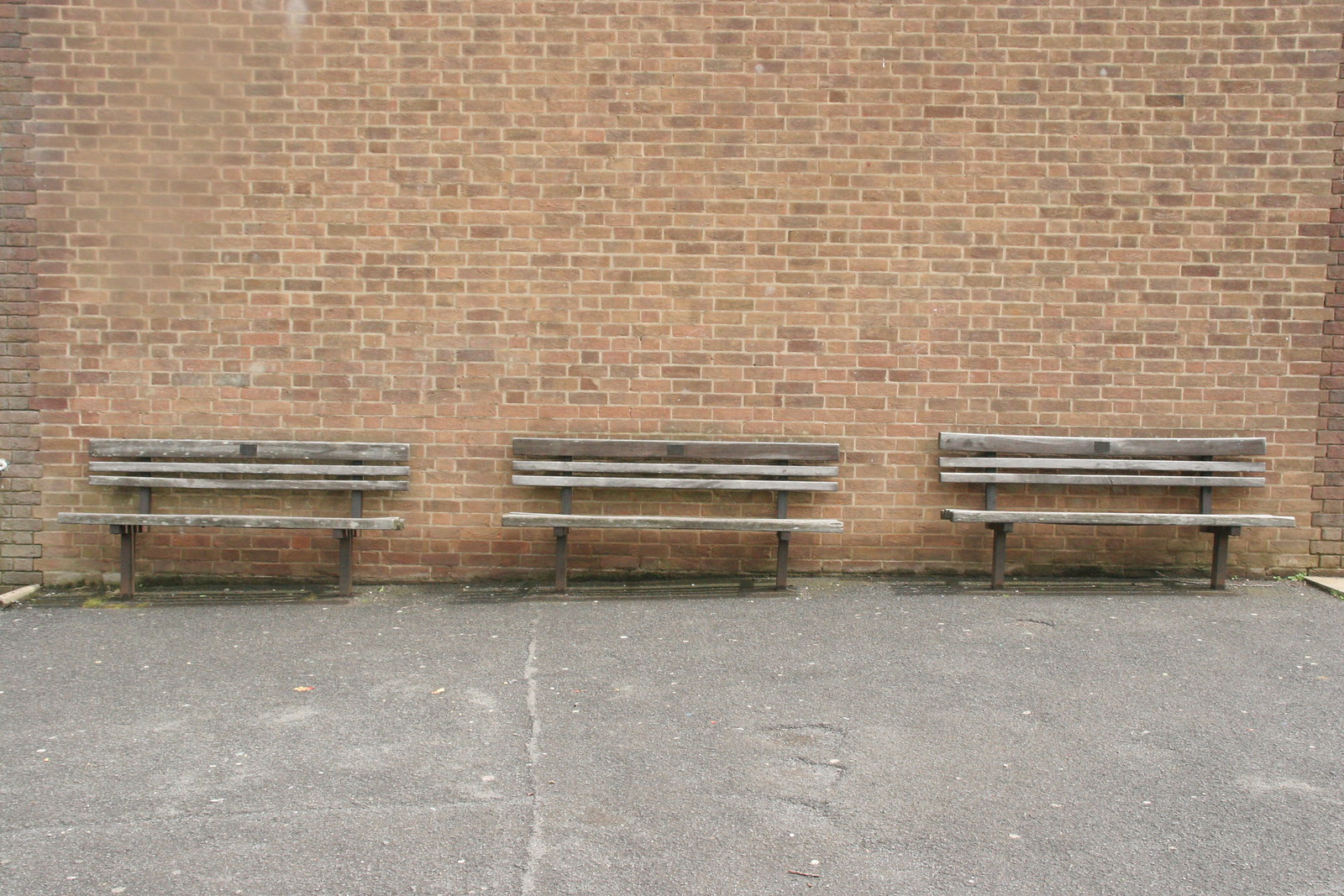The image depicts a row of three aged, wooden park benches positioned against a medium brown and light reddish-brown brick wall with white grout. Each bench, appearing distressed and weathered, has three wooden slats for the backrest and a single plank for the seat, all supported by metal bars on the sides. Notably, each bench features a small metal plaque on the backrest. The ground in front of the benches is gray concrete, marred by a visible, white crack running from the front towards the wall, just right of center. Additionally, there seems to be tan cement trimming in sections of the ground. Subtle details, like potential mold along the bottom edge of the wall and general dilapidation, give the scene an intentional, rustic charm.